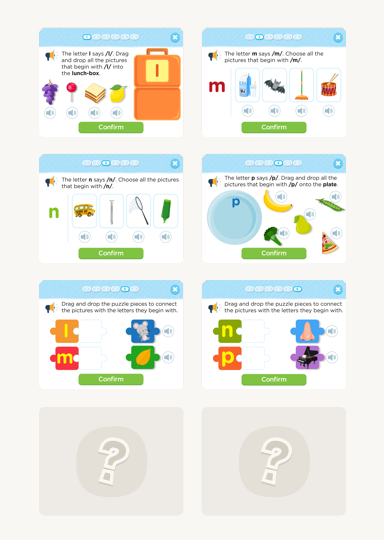This image features two side-by-side screenshots from a phone. Both screenshots display a series of small images arranged in a vertical sequence against a white background, with a light blue banner at the top. Unfortunately, the font is too small to read, but the visual elements are discernible through their colorful and varied designs.

In the left screenshot:
1. The first image features a simplistic, orange drawing of an upright carry-on suitcase against a white background.
2. The second image shows what appears to be a cluster of grapes, a red balloon, a yellow pitcher, and a small stack of wood.
3. The third image includes a green letter, a small illustration of a school bus, and, at the bottom, four puzzle piece-like shapes with the lower left piece being red and displaying a yellow letter "M".

In the right screenshot:
1. Similar to the left, the top section also houses simplistic drawings and assorted items within a white box bordered by a light blue top edge.
2. The images follow the same layout as the left screenshot, with three images arranged from top to bottom, each containing a randomized collection of small, colorful illustrations.

Overall, both screenshots exhibit an eclectic assortment of small, detailed images and shapes, spanning from practical objects like a suitcase and school bus to more abstract representations like puzzle pieces and letters.